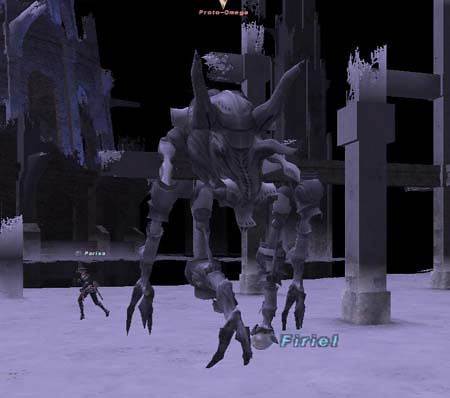This image is a dark, detailed screenshot from a video game depicting a dramatic scene with a towering, four-legged monster. The setting features a black background and a white floor, with steel beams rising up, some appearing split and collapsed. Center stage is a colossal creature, around 30 feet tall, with imposing horns on its head and elongated arms that reach down to the floor. The monster's legs bend like those of a crab, and it possesses large claws on both its arms and legs, which end in hooves split into threes. The name "F-I-R-I-E-L" is prominently displayed beneath the creature in blue text. Above the monster, in orange text, is a partially legible label that appears to spell "PROTOMEGA." The distant figure of a person, clad in dark armor and possibly in a stance of readiness or retreat, adds to the tense atmosphere. Scattered steel columns, some adorned with icicle-like formations, enhance the chilling, mechanical environment.